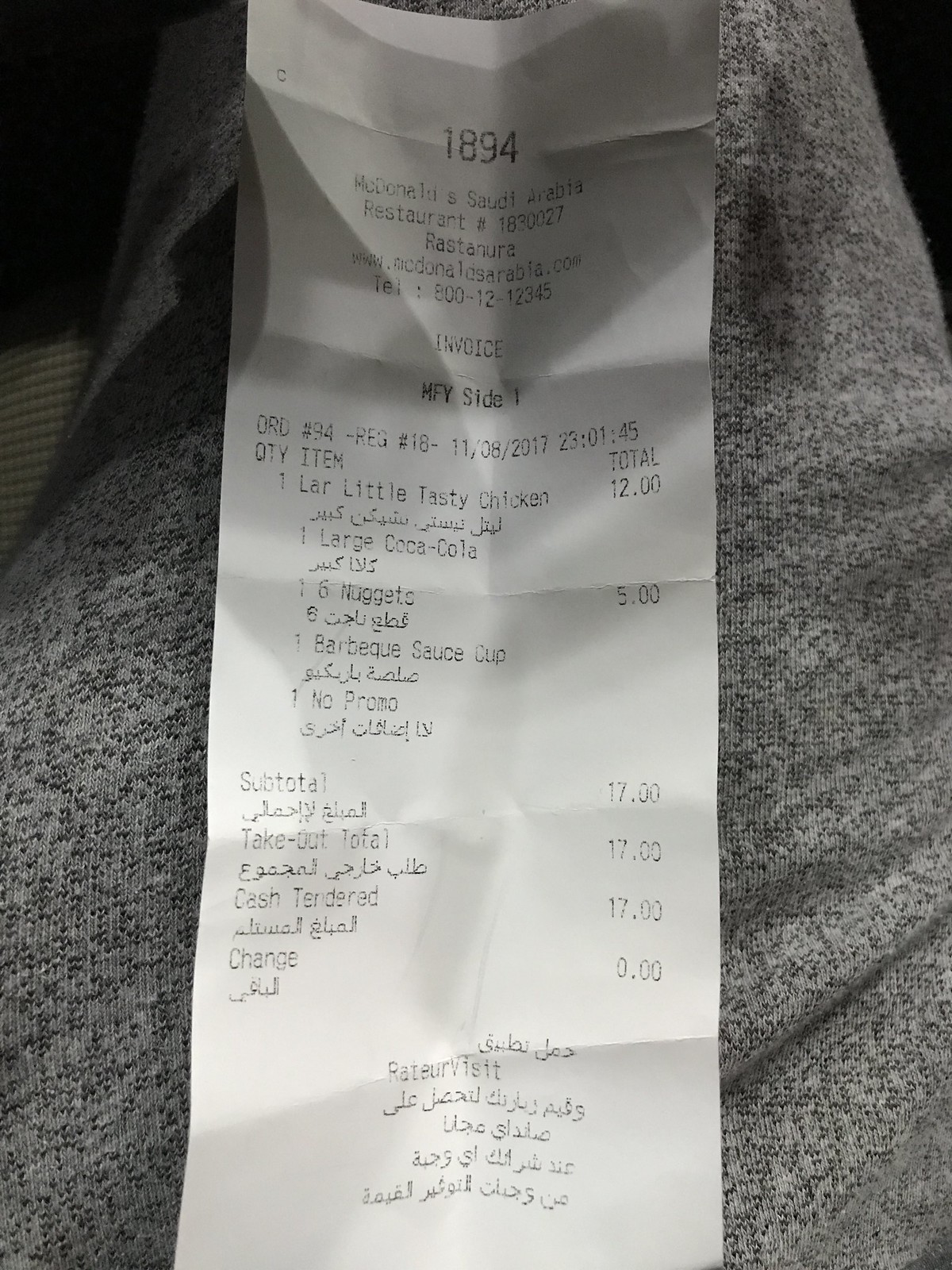The image depicts a crumpled McDonald's receipt from Saudi Arabia, laid out on a person's gray sweatpants-clad leg. Despite its creases from being folded, the receipt is legible and prominently displays the order number 1894 at the top. Below that, it reads "McDonald's, Saudi Arabia" followed by the restaurant number 1830027 and other establishment details. The listed items in the order are a large Little Tasty Chicken, a large Coca-Cola, a Six Nuggets, and a Barbecue Sauce Cup, with all the order details presented in both English and Arabic. The total amount is 17 units of the local currency. At the bottom of the receipt, there is additional information written in Arabic.